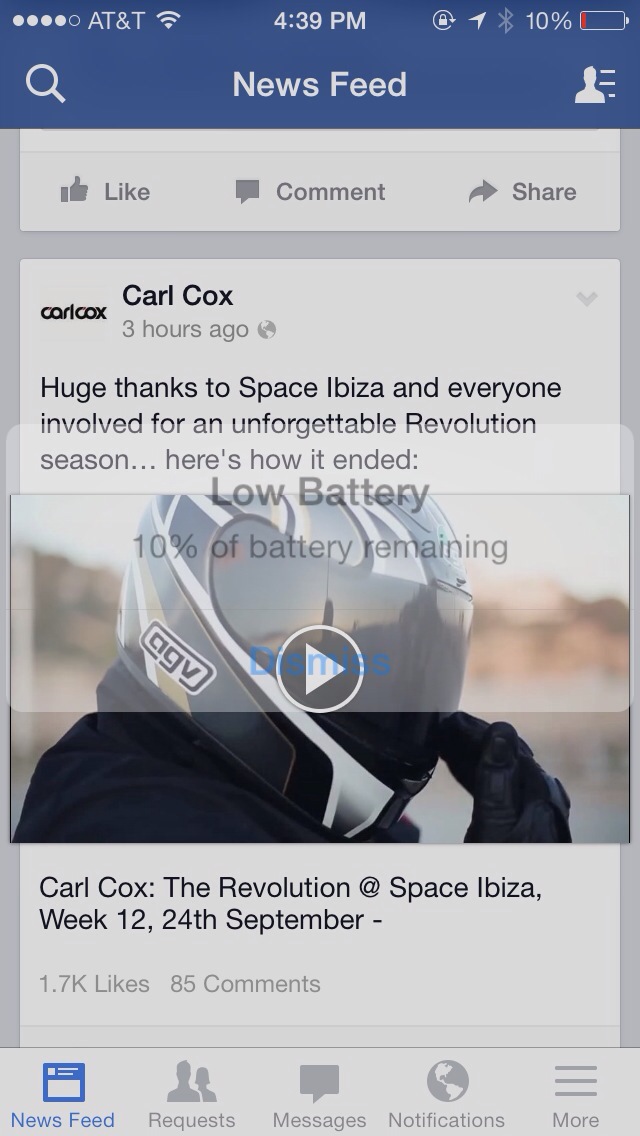This image captures a Facebook News Feed on a cell phone screen with AT&T as the network provider, showing the time as 4:39 PM and the battery level at a critical 10%, even generating a low battery warning pop-up. Below the status bar, the screen's main interface features a magnifying glass icon, the text "News Feed" at the center, and an icon to the right. The next row presents options for interacting with a post: "Like" with a thumbs-up icon, "Comment," and "Share" with an arrow icon. 

The central part of the screen displays a post by Carl Cox, timestamped three hours ago. The post reads: "Huge thanks to Space, Ibiza and everyone involved for an unforgettable revolution season. Here's how it ended," accompanied by a video thumbnail featuring a circular play button in the middle. In the background of the post, a faint prompt indicates, “Low battery: 10% of battery remaining.” Beneath the video, text confirms, "Carl Cox, The Revolution at Space, Ibiza, Week 12, 24th September," followed by engagement metrics showing 1.7K likes and 85 comments.

At the bottom of the screen, a navigation bar includes five icons labeled from left to right: News Feed, Requests, Messages, Notifications, and More.